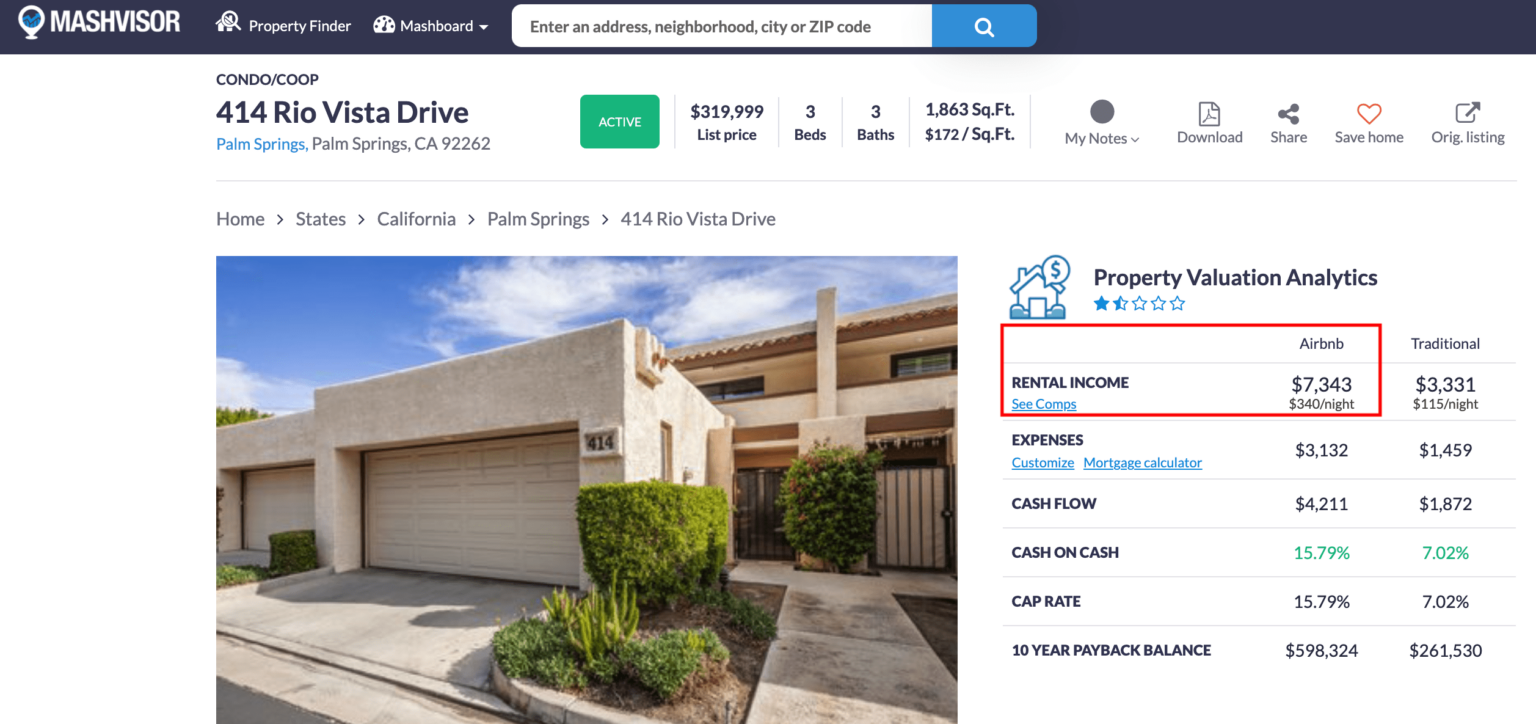This image showcases the MASHvisor website interface. At the top left corner, the MASHvisor logo is prominently displayed. Below the logo, there are two main options—"Property Finder" and "MASHboard." A search bar is located to the right of the "MASHboard" option, with a placeholder text that reads "Enter an address, neighborhood, city, or zip code." This indicates the website's function as a property search tool. 

The selected property is "414 Rio Vista Drive" in Palm Springs, California, 92262. To the left of the selected address is a photo of the property, providing a visual reference. To the right of the photo is a detailed description of the property’s income potential. The description is divided into six rows, with the first row highlighting rental income. Specifically, it notes that the Airbnb income is $7,343 per month, with an average nightly rate of $340.